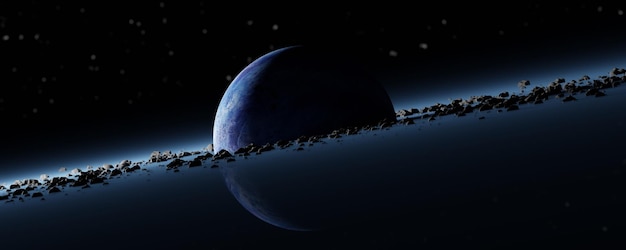The image appears to be a digital representation of a nighttime outer space scene. Dominated by a black, starry sky, the visual centerpiece is a partially illuminated planet, showcasing a striking contrast between its dark and light sides. Only the left side of the planet is visible, reflecting a soft light blue hue, while the right side remains shrouded in darkness. A distinctive diagonal line, resembling a ring or debris field, cuts across the center of the planet, extending from the lower left to the upper right. This line appears composed of scattered, floating rocks, contributing an additional layer of ethereal detail to this cosmic depiction. The interplay of light and dark elements combined with the scattered debris creates a captivating and surreal outer space tableau.